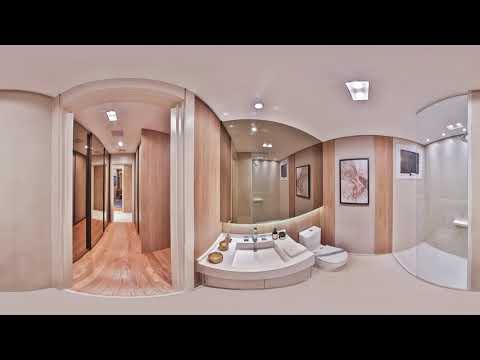The image depicts a luxurious and modern bathroom adorned in a soft peach color palette, with varying shades of peach creating a harmonious and elegant atmosphere. Central to the composition is a sleek sink, complemented by gold objects on the counter beside it. To the right of the sink is a low-standing toilet, adjacent to a peach-colored abstract picture on the wall. Further right, a large, curved shower with a pristine white interior enhances the space's contemporary feel.

The floor appears to be composed of tiles, adding a touch of texture and sophistication to the room. To the left of the sink, a doorway leads to a hallway characterized by light-colored wood flooring and walls, with one mirrored wall reflecting the opposite side, adding depth and dimension. The hallway appears somewhat circular, suggestive of 360 imaging which causes a warping effect, making elements of the room—including numerous arches and curves—appear stretched.

The bathroom also features a bathtub and a mirror centrally located in the image. The scene is framed by solid black borders at the top and bottom, accentuating the luxurious and well-thought-out design. The overall color scheme includes shades of soft peach, light pink, various tones of brown and tan, and touches of black and gray, creating a warm and inviting indoor space.